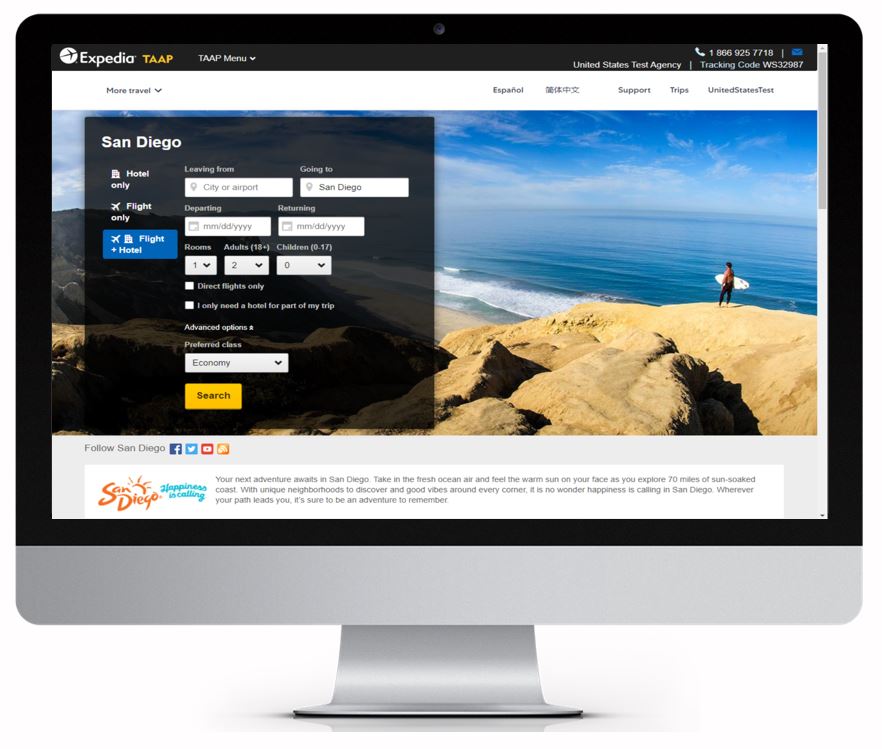The image, captured from a website, is set against a white backdrop and primarily focuses on a computer screen displaying a booking interface. 

### Header Section:
- **Top Left**: A white circle with a black plane flying diagonally to the top right, next to the "Expedia TAAP" logo.
- **Top Center**: The "TAAP menu" text in white, followed by a downward-facing white drop-down icon.
- **Top Right**: Text in white reading "United States Test Agency" followed by "tracking code WS32-967." Above this text is a white phone icon with the number "1-866-925-7718" to its right, and a blue envelope icon even further to its right.

### Navigation Bar:
- **Left**: The phrase "More Travel" in black, accompanied by a drop-down arrow.
- **Center**: Language options including "Español," and Asian characters (Japanese or Chinese), followed by icons for support and trips.
- **Right**: Text indicating "United States Test."

### Main Search Area:
- **Top Left**: A black box containing the text "San Diego."
- **Below "San Diego"**: White text stating "Hotel Only," a white airplane icon next to "Flight Only."
- **Below "Flight Only"**: 
  - A blue box featuring a white airplane icon and a piece of paper, labeled "Flight + Hotel."
  
### Input Fields:
- **Leaving From**: A white box for entering the city or airport
- **Going To**: A white box with a map icon and "San Diego" indicated.
- **Departing**: An input field for selecting the departure date.
- **Returning**: An input field for selecting the return date.
- **Rooms**: A dropdown with a default value of "1."
- **Adults**: A dropdown (default "2") with a note indicating ages 13+.
- **Children**: A dropdown (default "0") with age range 0-17.
- **Direct Flights Only**: A checkbox.
- **Additional Preferences**: Options for additional trip needs and advanced options.
- **Preferred Class**: A dropdown with "Economy" selected.
- **Search**: A yellow search button located on the lower right.

### Background Image:
- **Setting**: An oceanic landscape with a visible sky and rocky bottom right corner.
- **Figure**: A man standing on a rock, wearing a partially rolled-down black wetsuit, exposing his bare chest, holding a white surfboard.

The overall layout combines navigational elements, input fields for booking travel, and a scenic background, encapsulating a typical online travel booking interface.